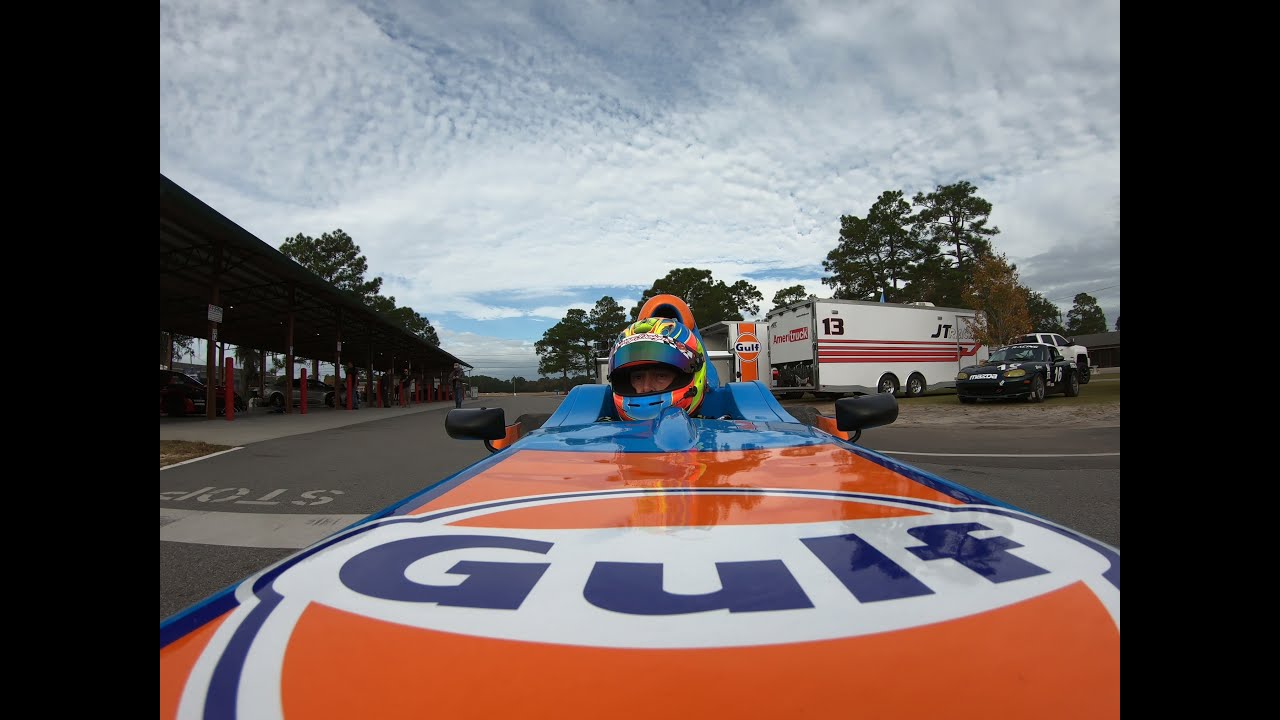The image captures an F1-style race car from a GoPro-like perspective, mounted at the front of the vehicle and facing back towards the driver. The car, predominantly orange and blue with a prominent Gulf logo in blue text circled in white, stands out vividly. The driver, sporting a multicolored helmet adorned with shades of orange, white, green, and blue, is seen clearly in the open cockpit without any roof or protective casing, emphasizing the high-speed, high-risk nature of the sport. In the background, there's an assortment of vehicles including trailers, trucks, and another racing car, alongside a few trees and a cloudy sky, giving a sense of a bustling race track environment. A large truck marked with the number 13 and a Gulf-branded truck also feature in the scene, adding to the atmosphere of a professional racing event.